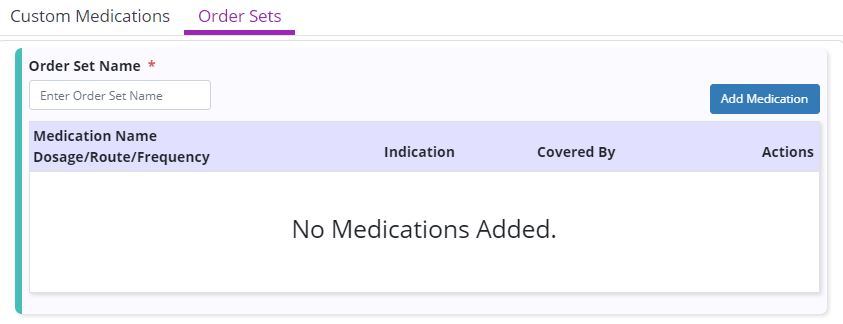This image captures a detailed page dedicated to custom medications. At the top, the title "Custom Medications" is prominently displayed, followed by "Order Sets" in bold purple font, underlined with a thick purple line. Two faint gray horizontal lines run across the top of the page beneath this header.

On the left side, the section labeled "Order Set Name" is marked with a red star, indicating a required field. Below it, a box prompts users to "Enter Order Set Name." At the end of this line, a blue button with white text reads "Add Medication."

Moving down, there's a rectangular section. The top of this section is highlighted in a purplish shade, while the bottom remains plain white. This section includes fields titled "Medication Name," "Dosage," "Route," and "Frequency." Below these, there is a large blank space. In the middle, another field labeled "Indication" is present, followed by spaces for "Covered By" and "Actions." At the bottom, an announcement in large font declares "No Medications Added."

The left side of the rectangular section is bordered by a teal-green and blue line, adding a distinctive visual element to the page.